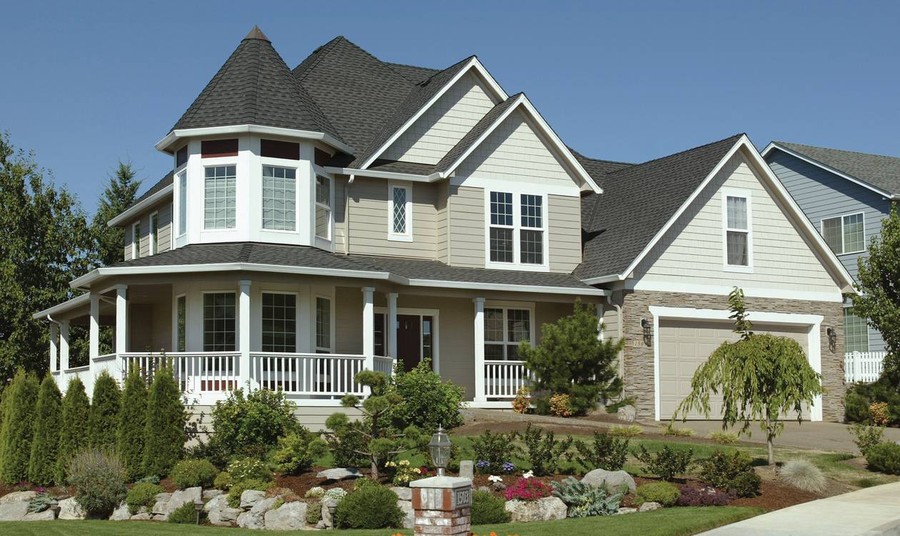The image showcases a stunning, contemporary house with a light gray and tan exterior, accented by a dark charcoal gray rooftop. A distinctive feature is its white wooden porch, which wraps around the front and left side of the house, supported by arches and white railings. The garage door on the right side of the house is a cream or light beige color, framed in white. The house is nestled in lush landscaping, with a variety of trees and substantial bushes surrounding the front, alongside neatly trimmed green shrubs and red flowers. Gray stones outline a mulch-covered garden, and a stone arch with the house address and a glass light on top is situated on the lawn. The backyard is framed by tall trees, while the front yard features hedge-like green trees and neatly arranged plants, adding a vibrant touch of green. The sky is a flawless blue, enhancing the overall charm of the house, which is set in a neighborhood with a neighboring light blue house to its right.